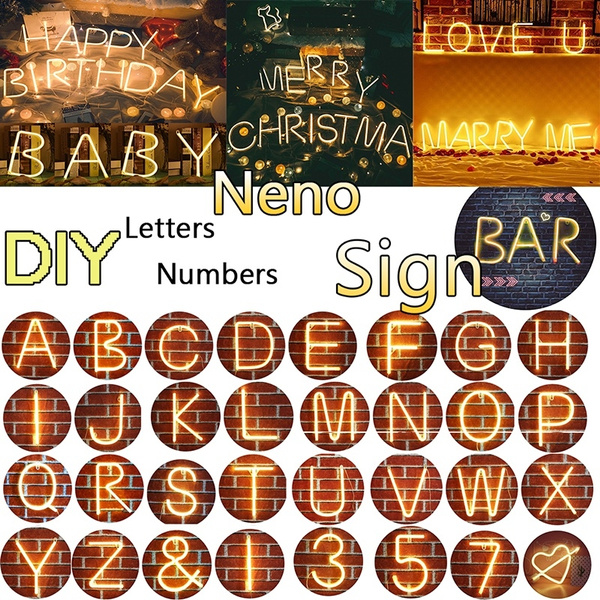The advertisement showcases a series of customizable neon signs available for purchase. At the top, the image displays three example designs: one reading "Happy Birthday Baby" in bright white lights, another stating "Merry Christmas" also in white lights, and a third displaying "Love You, Marry Me" in a light yellow hue. Each message is set against a dark, red brick wall background, emphasizing the glow of the neon letters. Below these examples, the ad mistakenly spells "Neon" as "Nino" but prominently highlights “DIY Letters & Numbers” in yellow and gold bubble letters. Toward the middle, there is a circle labeled "Bar," filled with black bricks and illuminated by neon. The bottom section of the advertisement features a comprehensive display of all available neon letters and numbers, arranged in four rows of eight. This includes: A-H, I-P, Q-X, Y-Z, along with additional characters like the ampersand (&), numbers 1, 3, 5, 7, and a heart with an arrow through it.